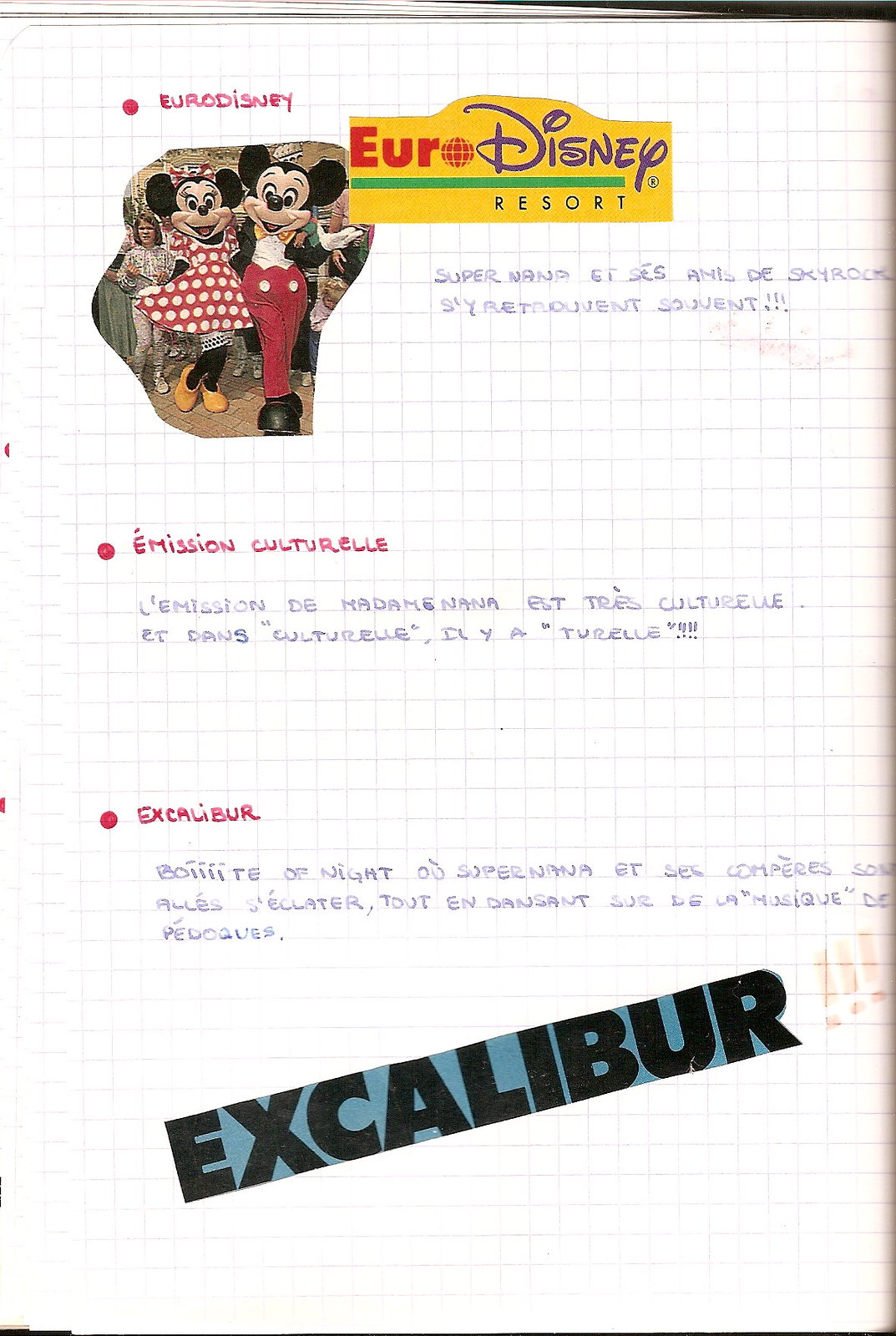This image depicts a scrapbook page with a grid-lined background. At the very top, the page features a red bullet point followed by the handwritten word "Euro Disney" in red ink, next to a pasted cutout of Mickey and Minnie Mouse with people in the background, and the Euro Disney Resort logo. Beneath this image, there is some fine handwritten text in French, difficult to read due to its size and faded nature.

Moving down the page, there's a second red bullet point followed by the word "Emission Culturelle" in red text, with more detailed black handwritten French text beneath it. Further down the page, another red bullet point appears, with the word "Excalibur" written in red, followed by additional handwritten French text. At the very bottom of the page, another cutout features the word "Excalibur" in black text on a blue background, embellished with three exclamation points written in a highlighted color. The colors on the page include red, white, black, yellow, green, purple, and blue. The overall layout and style of the page suggest it is casually made and unprofessional.